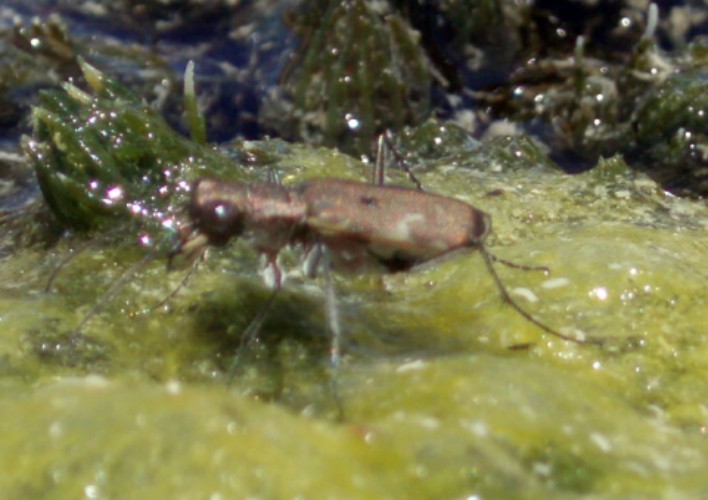In the close-up photograph, we see a brownish insect with distinctive, large, domed eyes and several slender, angular legs. The insect features prominent antennae emerging from the front of its face. It is positioned upright, seemingly walking on a green, slimy, and wet-looking surface that could be some sort of moss or algae, suggestive of a damp or watery environment. The insect's body, approximately three inches long and two inches high, has a camouflage-like pattern with brown and gold splotches, enhancing its grotesque and somewhat "ugly" appearance. The background includes various shades of green, likely plants, and some blue-tinted water, indicating a natural, possibly creek-side habitat.